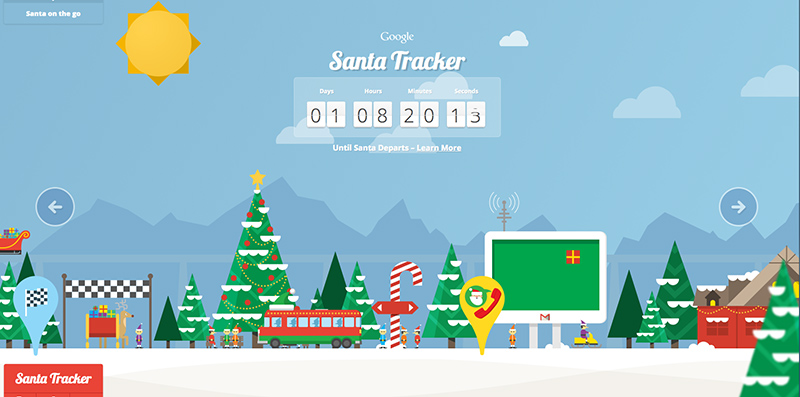The screenshot depicts the Google Santa Tracker interface with a festive, holiday-themed design. The background is a light blue adorned with clouds and snow-capped mountains at the bottom. Dominating the scene are various Christmas icons, contributing to the overall Christmassy feel.

In the top left corner, there is a button featuring white text alongside a geometric sun image. Centrally positioned in the header is the "Google Santa Tracker" logo, beneath which lies a countdown timer that displays the number of days, hours, minutes, and seconds remaining until Christmas, updating continuously.

Scattered across the scene are vibrant Christmas trees decorated with ornaments and topped with stars, creating a joyous atmosphere. A red and green trolley adds to the festive color palette. Snowy evergreens and a backdrop of snow cover the lower section, further enhancing the wintry theme. 

Central navigation is facilitated by forward and back arrows on either side of the screen, allowing users to explore additional features. An intriguing element, possibly a sleigh with a satellite, is present as well. To the left, a checkered race-like structure features a reindeer carrying presents, with the "Santa Tracker" logo positioned in the bottom left corner, integrating seamlessly into the overall cheerful design.